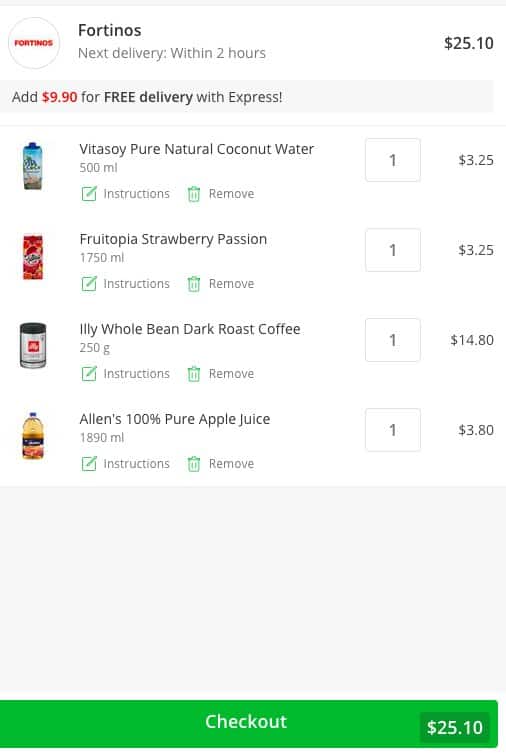This image is a screenshot of a section from an online shopping website for Fortinos. The screenshot, cropped for brevity, has no visible web browser details and is of low quality, with a slight blur that still permits readability. Dominating the top of the image is the Fortinos logo: a white circle with the word "Fortinos" in red inside it. Adjacent to the logo, the name "Fortinos" is also written in black text, with a grey subheading below it stating "Next delivery within 2 hours."

In the top right corner, the total cost of the order is displayed as $25.10. An alert message indicates that an additional $9.90 is needed for free delivery through Express. This order consists of four beverage items: coconut water, a strawberry drink, roast coffee, and apple juice. At the bottom of the screenshot, there is a green "Check Out" button, inviting the user to finalize their purchase.